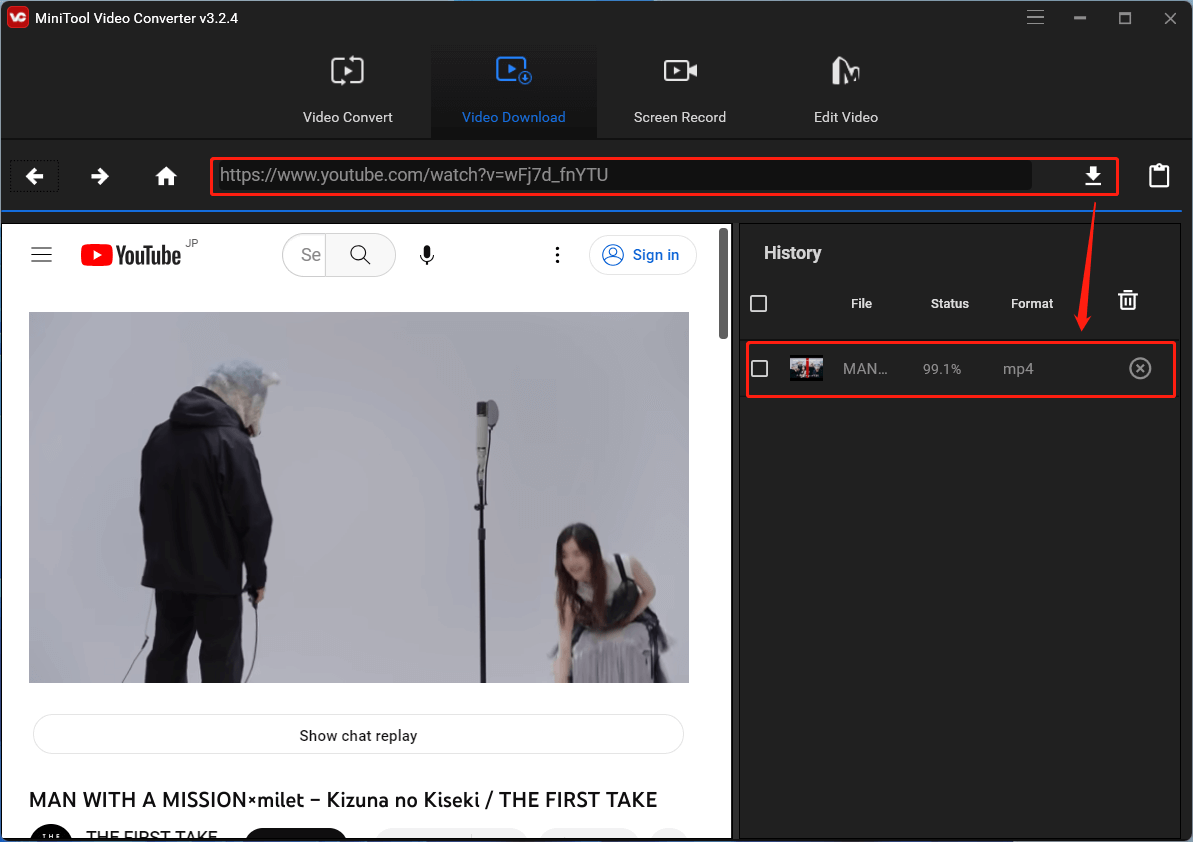This image appears to be a screenshot from a software application called MiniTool Video Converter V3.2.4. The app interface is primarily focused on video downloading and converting functionalities. The screenshot shows a small red icon labeled "VC" at the top. 

In the center of the interface, there's a prominent visual symbol composed of two curved arrows that form a circular shape, with a play button triangle in the middle, representing the video conversion feature. Underneath this symbol, different functionalities are displayed as tabs: 'Video Download' (highlighted in blue), 'Video Convert' (in white), 'Screen Record' (in white), and 'Edit Video'.

On the right side of the screen, there's a YouTube link highlighted and circled in red, indicating an active video download process. Accompanying this is a download icon along with several status indicators such as 'History', 'File', 'Status', and 'Format'.

Further down, there is a thumbnail of the YouTube video currently being downloaded. The video features an unusual scene: a man wearing a horse head and presenting his back to the viewer while a woman in a Bavarian dress is kneeling. The video is titled “Man with a Mission, XMILET, Kizuna No Kiseki, K-I-S-E-K-I” and is part of 'The First Take' series.